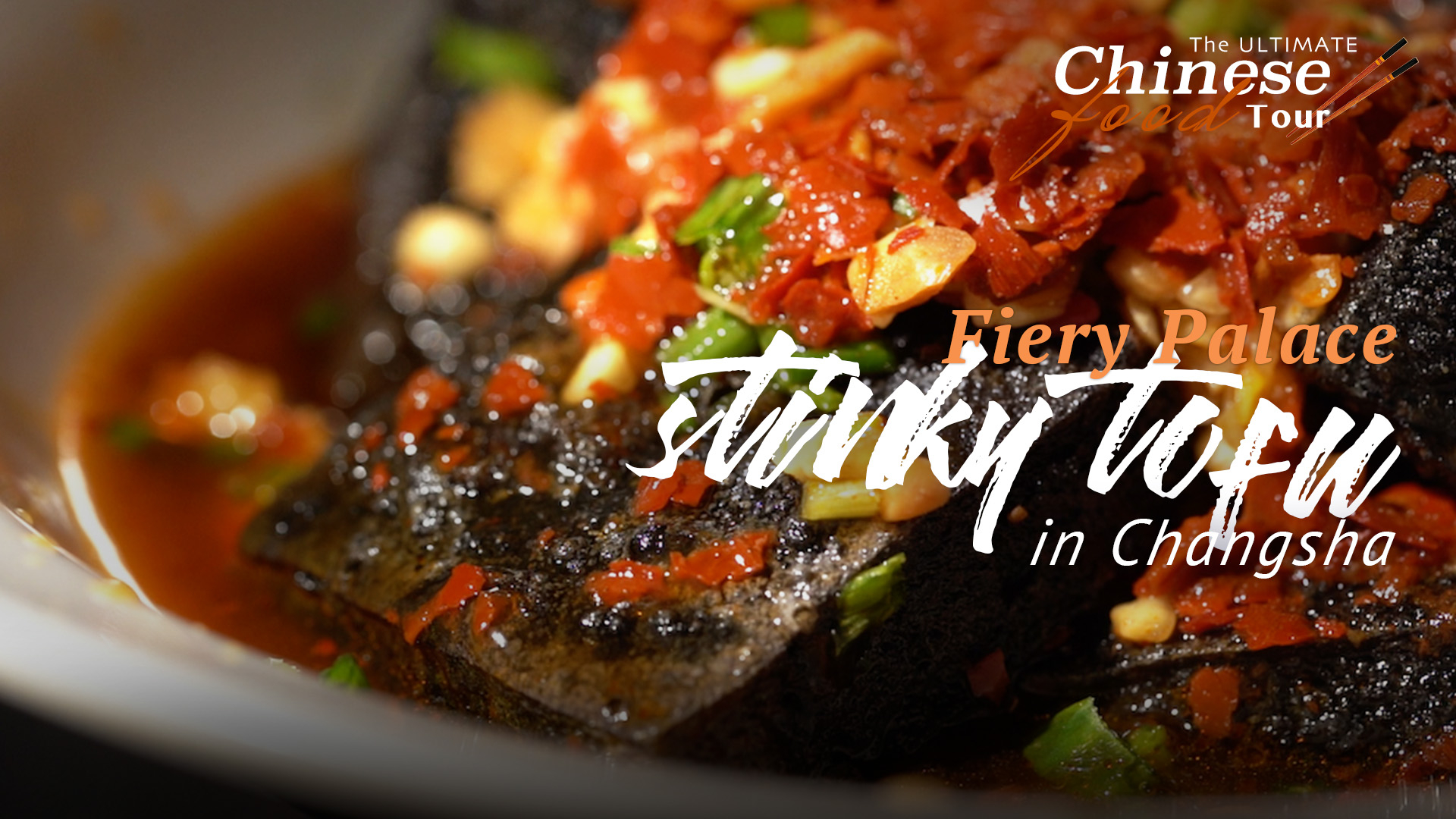**The Ultimate Chinese Food Tour: Fiery Palace Stinky Tofu in Changsha**

Dive into the vibrant flavors of Changsha with the renowned dish, Stinky Tofu from Fiery Palace. This captivating ad showcases a savory concoction that resembles succulent cuts of steak, but is actually aromatic and richly seasoned tofu. The dish bursts with color and zest, featuring a medley of sautéed and seasoned vegetables, including bright red tomato slices and a variety of green and yellow vegetables. The tofu, affectionately and intriguingly named "Stinky Tofu," promises an unforgettable culinary experience, tantalizing your taste buds with its juicy and enticing presentation. Whether a tofu lover or a curious food explorer, this dish invites you to savor the unique and adventurous flavors of Changsha's culinary landscape.